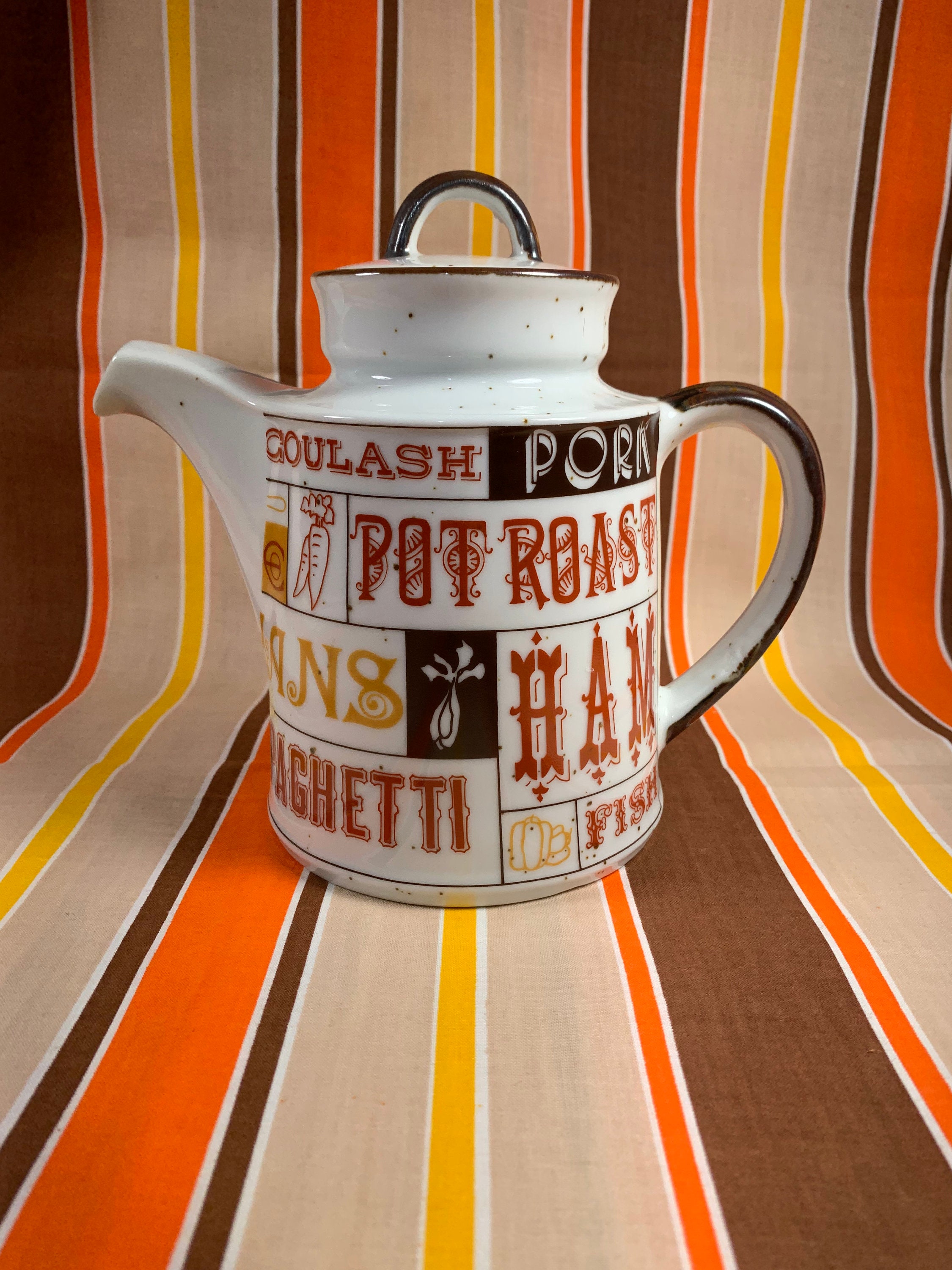This close-up photographic image captures a large white ceramic teapot with a brown handle and a matching brown lid. The teapot is adorned with orange text listing foods such as "goulash," "pork," "pot roast," "ham," "fish," and "spaghetti." Beside the text, there are small graphic illustrations of food items like carrots, a pepper, some root vegetables, and a piece of fish. The teapot, which also features a spout, is placed on a piece of fabric. The fabric is richly colored with stripes of orange, yellow, black, and various shades of brown, adding a vibrant backdrop to the scene. The cloth appears to be draped both behind and beneath the teapot, creating an aesthetic setting that suggests this photograph might have been taken with the intention of selling or showcasing the teapot.